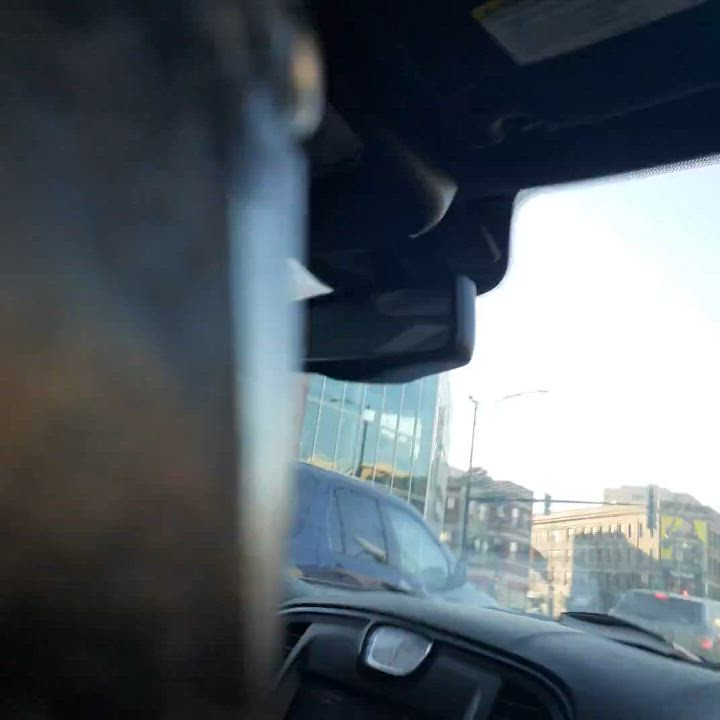This photo, taken from the backseat of a black car, captures a detailed urban scene through the front windshield. Dominating the left half of the image is a blurry, dark shape likely the driver's seat or headrest. The right half showcases the car's dashboard, including an illuminated white clock. Centered in the frame hangs the rearview mirror, descending from the car's ceiling. Just beyond the dashboard, the image reveals a street peppered with vehicles, including a black SUV and a brown SUV. The cars appear stationary, halted by visible traffic lights, suggesting the car wasn’t in motion at the moment. Framing the scene outside, several low-rise, multi-windowed brick buildings stretch along the street, lending an office or apartment vibe to the urban setting. The sky above is predominantly white with a tinge of blue, indicating a bright, cloudless day.